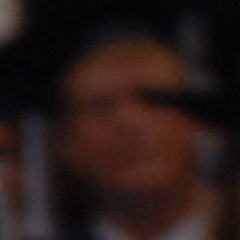This image appears to be a cropped section of a photograph, rendering it quite enigmatic. Dominated by darkness and intense blur, the content is almost indiscernible; however, it seems to depict a human face, potentially a man's, characterized by light skin. The face is directed towards the camera, devoid of facial hair, and potentially features short, light-colored hair. A white or light-toned collar is faintly visible, providing some contrast. On the right side of the image, a darker object intrudes into the frame, partially obscuring one of the person's eyes and adding to the overall obscurity.